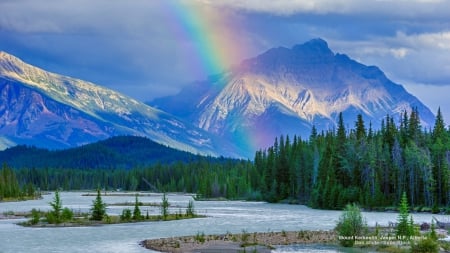This is a detailed photograph of Mount Kirkuslin in Jasper National Park, Alberta, Canada. The image showcases a stunning mountain range with snow-capped peaks and sharply angled rocky surfaces set against a sky heavily adorned with clouds. The sunlight illuminates a slice of the mountains, enhancing their blue and white hues. A vibrant rainbow descends through the photograph, seemingly arising from behind a tree line in front of the mountains and dissipating into the dense forest below. In the foreground, a large body of water, possibly a river, stretches out, displaying ripples and reflective surfaces that mimic the look of ice or small white caps. This waterway is dotted with several sandy islands, each sparsely populated with isolated pine trees. The right side of the image features a tall hill covered in green pine trees, and in the distance on the left, a lower, tree-covered hill fades into the background. Tiny, unreadable text in the lower-right corner of the image serves as a descriptive note. The overall scene is one of serene natural beauty, combining elements of land, water, and sky in a harmonious landscape composition.